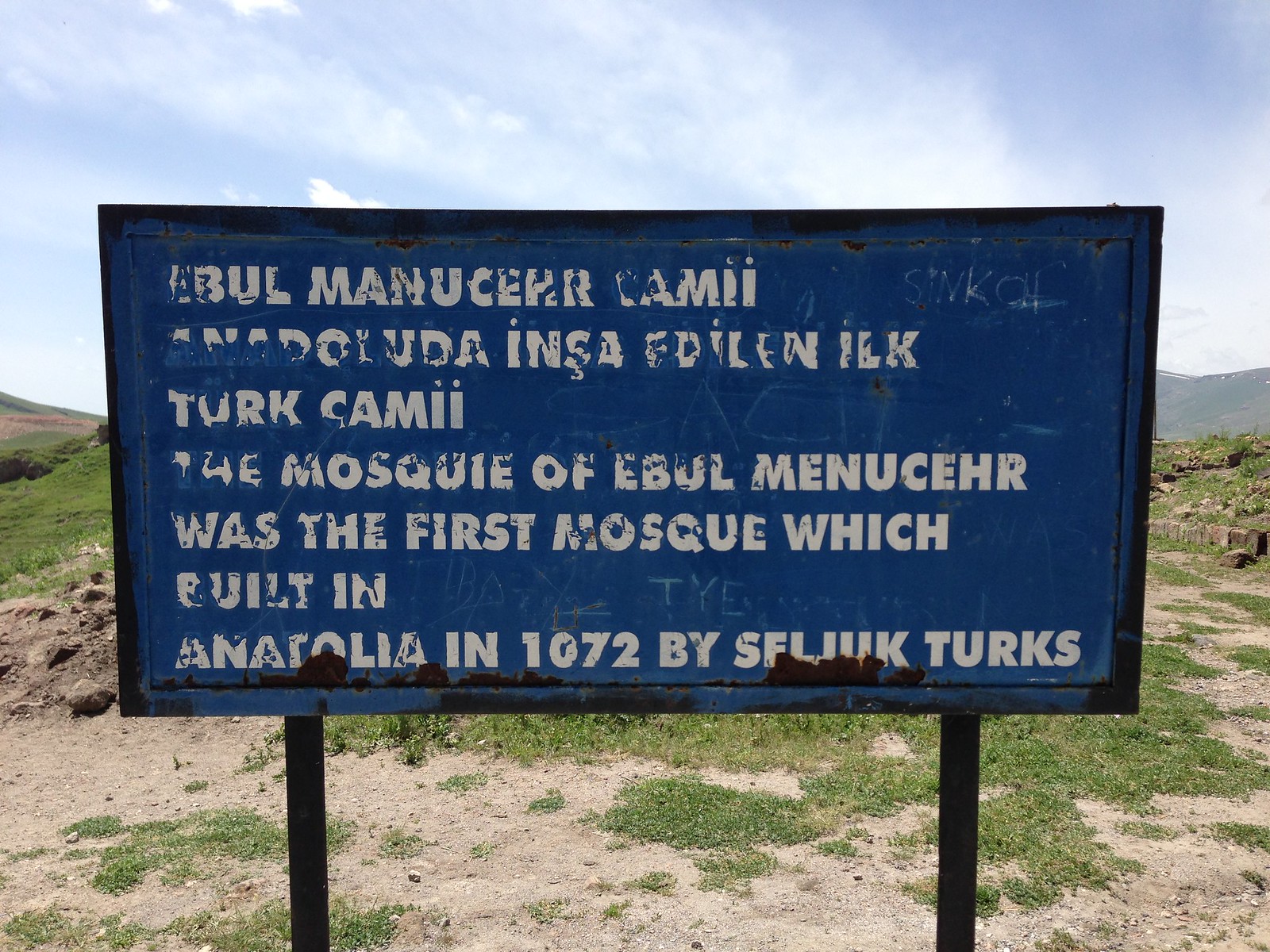An outdoor scene captured during the daytime shows a historical location with a prominent blue sign at its center. The sign is housed in a black metal frame with two supporting posts on either side. The sign bears white text displaying “Abu’l Manusepur,” among other less legible details, mentioning it as the site of the first mosque built by Turks in Anatolia in 1072. Encircling the sign, a rugged landscape unfolds with sandy, grassy patches and scattered rocks. In the distance, a range of mountains and undulating hills provide a scenic backdrop. Above, the sky is a soft blue, generously speckled with white clouds, adding depth and atmosphere to this outdoor historical setting.